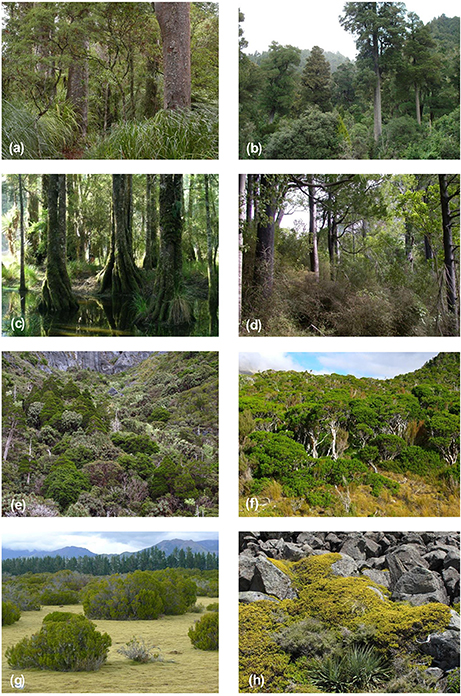The image is a collection of eight distinct outdoor photographs arranged in two columns, with each photo labeled from A to H. The first column contains images A, C, E, and G, and the second column contains images B, D, F, and H, with each label in the lower left corner. 

*Image A*, positioned at the top left, shows a lush forest scene with brown tree trunks and green leaves, accompanied by some bushes.
*Image B*, at the top right, presents a forest canopy with the tops of numerous trees, highlighting one particularly tall tree rising above the rest.
*Image C*, directly beneath A, features a swamp with trees standing in shallow water, their trunks appearing twisted or braided.
*Image D*, directly beneath B, displays more tree trunks and bushy vegetation, characterized by scrubby, brown underbrush.
*Image E*, below C, offers a valley view with an elevated perspective, looking down upon a dense treetop canopy amidst the landscape.
*Image F*, underneath D, also captures a valley scene from an elevated angle, showcasing a canopy of green treetops.
*Image G*, at the bottom left, depicts a transition from a foreground of dirt and green bushes to a middle ground with more foliage, culminating in distant trees and faraway mountains.
*Image H*, located at the bottom right, features a terrain of gray stones covered in green moss.

All photographs appear to be taken during daylight, depicting natural, wooded environments from either an elevated vantage point or a standing perspective. The color palette predominantly includes shades of green, brown, black, yellow, off-white, and beige, suggesting a consistent geographical region across the scenes.